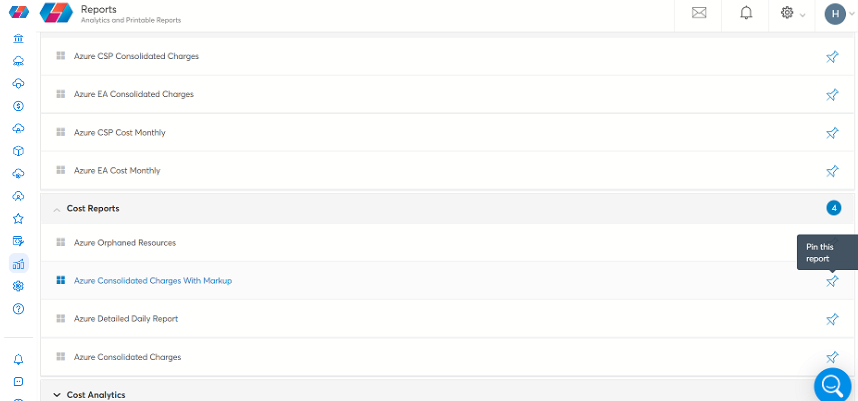This detailed screenshot captures the interface of a complex management dashboard. In the upper left-hand corner, the screen prominently displays the text "Reports," "Analytics," and "Printable Reports," hinting at the functionalities available to the user. On the upper right-hand side, there is a utility bar featuring a series of icons: a mail button for messages, a notification symbol for alerts, a settings button for configuration options, and a profile icon marked with the letter "H."

Directly below these elements, the interface is divided into several hierarchical sections. The top section is labeled "Azure CSP Consolidated Changes," followed by three other similarly structured subsections. Continuing downward, the next segment is titled "Cost Reports," which contains four more items before transitioning to another section labeled "Cost Analytics." However, the text in the subsections appears somewhat small and difficult to distinguish clearly.

On the left side of the interface, a vertical toolbar is populated with various icons representing different functionalities: a dollar sign, a box, a star, a settings icon, a help button, and another notification bell. Each icon is neatly aligned, assisting users in navigating through the dashboard. Finally, in the bottom right corner, a blue circular button with a white magnifying glass icon signifies the search function, providing an accessible way to explore further information within the dashboard. This layout, both comprehensive and intricate, emphasizes the dashboard's utility in managing and analysing a wide array of reports and data.